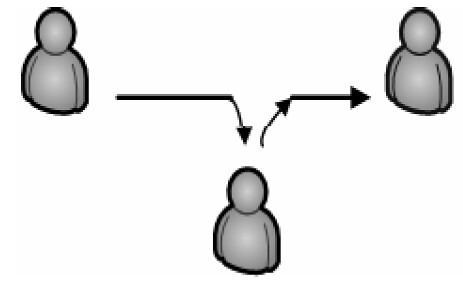The diagram features a sequence of three identical human-like figures, each represented by a simplistic, gray, waist-up icon reminiscent of the classic MSN logo. Each figure is outlined in black. The layout starts with a figure on the left side, with an arrow extending rightwards and then downwards, connecting to the second figure located at the lower part of the diagram. From this middle figure, another arrow points upwards to the center, directing to the third figure positioned on the right side. This final figure is linked by an additional arrow originating from the second figure. In summary, the diagram demonstrates a flow of movement between three identical icons through a series of directional arrows.